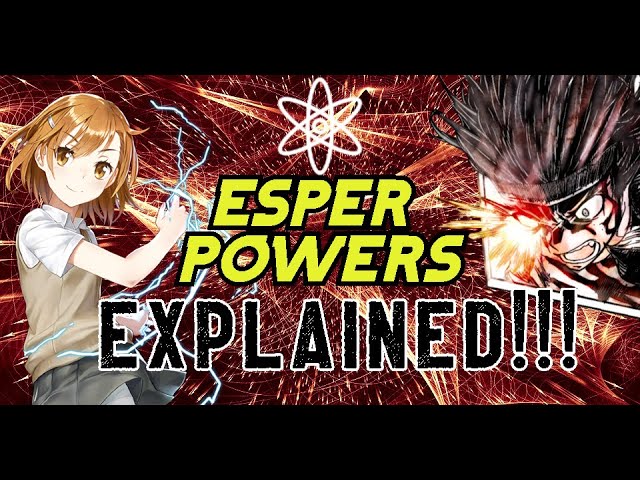In the image, two distinct anime characters occupy the scene. On the left side stands a young girl with light brownish-red hair that falls just below her jawline, framing her pale, white face. Her large brown eyes are wide open, conveying a sense of determination. She is dressed in a short-sleeved white shirt topped with a light brown plaid vest, paired with a black skirt. Her body is angled to the right, but her head faces forward. One arm is extended outward, and from her fingers emerge bright blue lightning bolts, hinting at her supernatural abilities.

To the right, a monstrous figure draws attention with its grotesque features. This character has black, spiky hair resembling a porcupine's quills and a shadowed, menacing face dominated by its wide-open, white eyes with black pupils. One of its eyes appears to be exploding, gushing red blood in all directions. The creature's mouth is agape, as if screaming, set against a chaotic background of dark red explosions and fiery sparks.

Centrally placed in the image is a large nuclear symbol, surrounded by three ovals, underscoring the theme of destructive power. Below this symbol, striking yellow text with a black outline reads "ESPER POWERS," and beneath that, black text with a white border declares "EXPLAINED!!!" The overall scene is framed by thin black bars at the top and bottom, lending the impression of a YouTube thumbnail or an eye-catching advertisement.